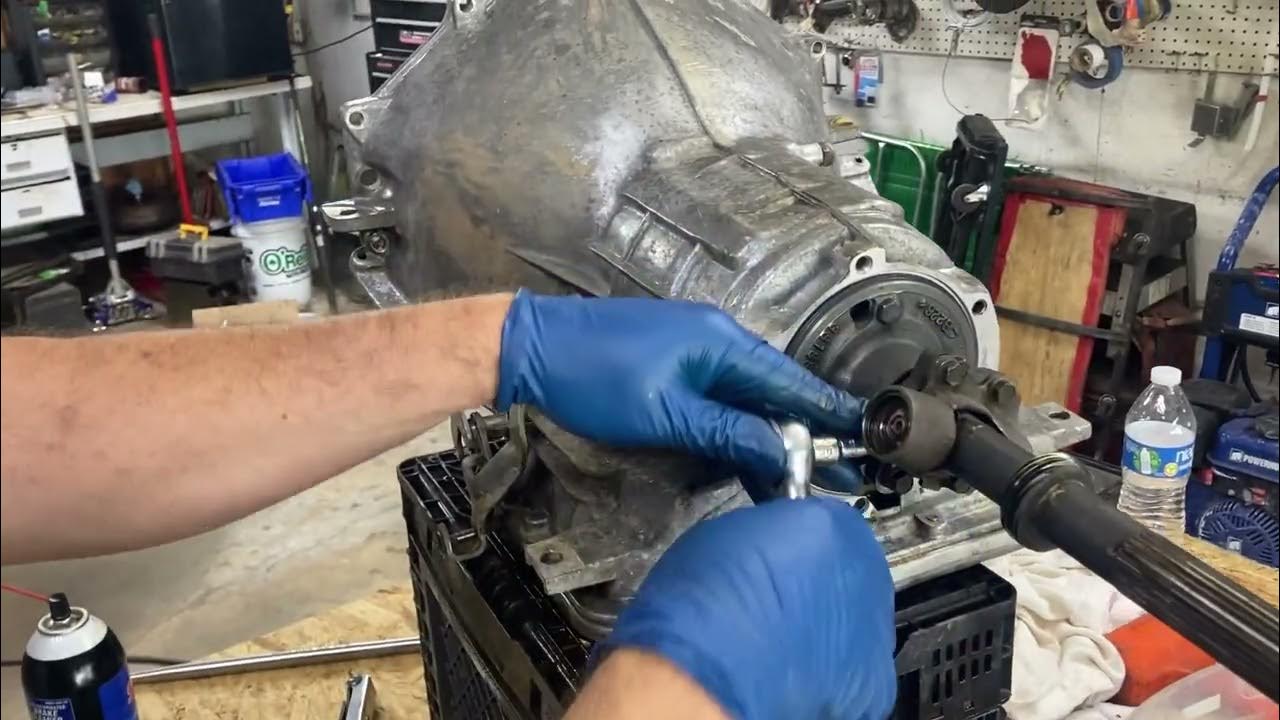The image captures a detailed scene of a mechanic diligently working in a cluttered garage. Central to the photograph is a silver piece of a car motor, which tapers as it extends towards the camera. At its wider end, there is a black cylinder with a long, black rod protruding bottom right. The mechanic's hands, wearing blue gloves, are working with a socket wrench on this motor component, specifically targeting the black cylinder. His left arm extends straight across the frame, while his right wrist and glove are visible holding the wrench.

The background of the garage is filled with a variety of tools and equipment. Car parts hang from the walls, and to the right are ladders, stools, and sliders. The left side of the image features more tools, a white table cluttered with metal products, and shelves with various items, including toolboxes and cans. Notably, a white and blue double-stacked bucket is situated in front of this table. A water bottle, a can of lubricant with a white top, and a cup branded with "O'Reilly's Auto Parts" are also visible on different surfaces. Overall, the scene portrays the mechanic's focused efforts amidst a densely packed garage, rich with the assorted paraphernalia typical of an industrious workspace.